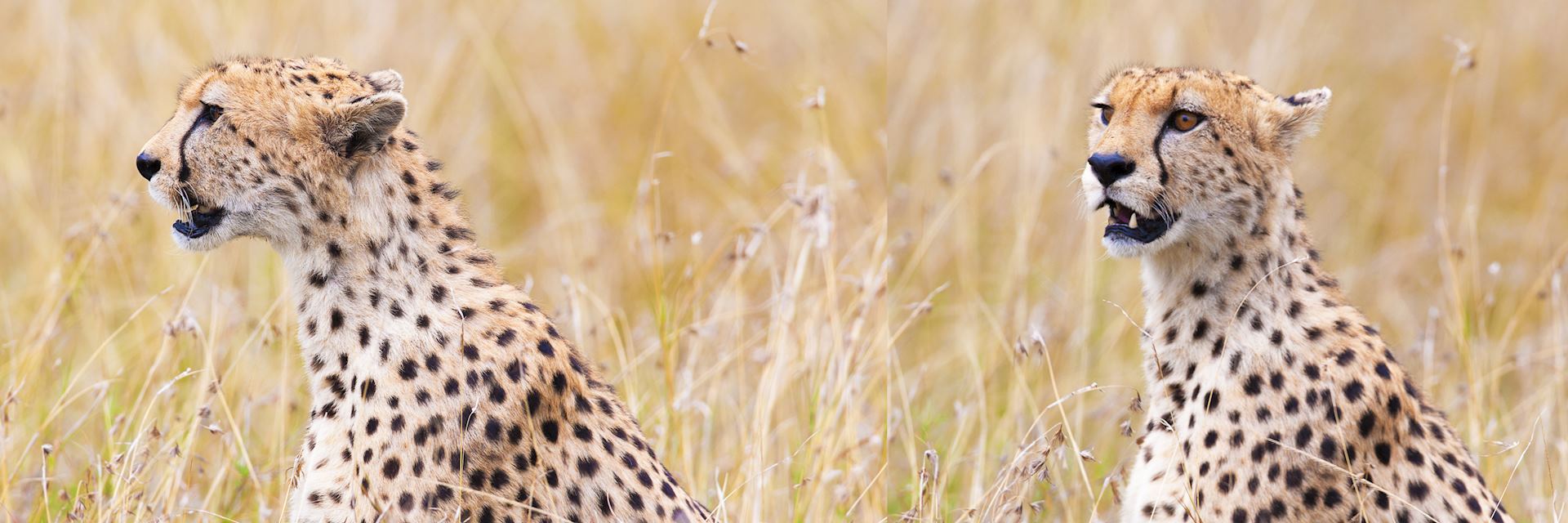In these two juxtaposed images, we see a pair of cheetahs set against the backdrop of an overgrown grassland, filled with tall, yellowing weeds typical of such habitats. The first image on the left captures a cheetah with its body and gaze directed to the left, partially camouflaged by the tawny grass which mirrors the cheetah's spotted fur. This feline appears vigilant, surveying the area. The second photo on the right provides a closer, more detailed view of the other cheetah, which has turned its head towards the camera. This cheetah's brownish-red eyes are clearly visible, along with distinctive facial markings—a brown streak descending halfway down its nose and a black line running from the inner eye to the corner of its mouth. The animal's fangs are noticeable, especially the sharper, slightly larger left fang. Both cheetahs are positioned amid shades of tan, brown, black, yellow, and green, emphasizing the natural setting far removed from human presence. The cheetahs sit with an air of alertness, their short ears slightly tilted back, as if attuned to the sounds of the wild around them.